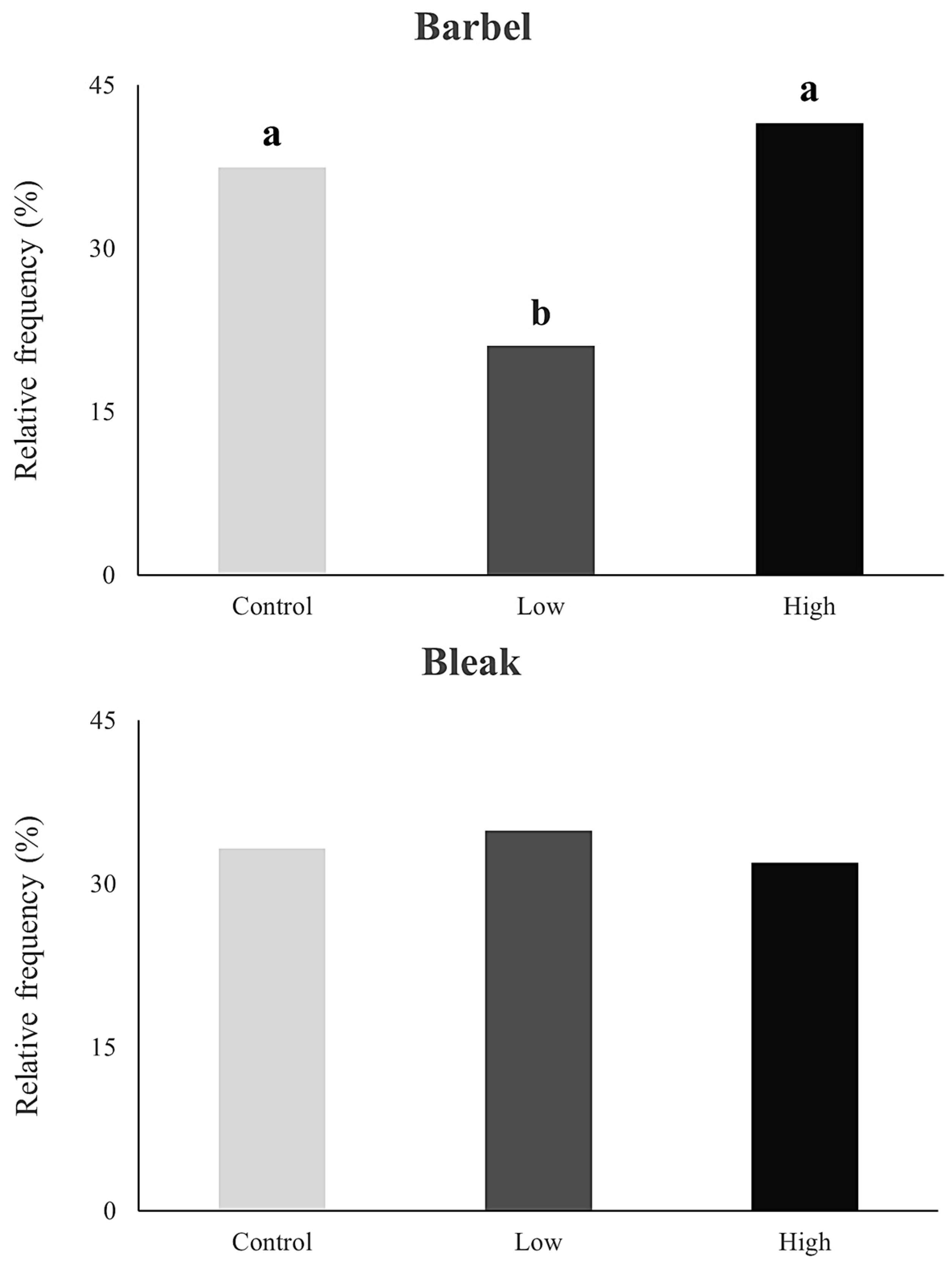The image consists of two distinct graphs stacked vertically. The top graph, titled "Barbell" in bold, black lettering, illustrates relative frequency values ranging from 0 to 45 on the vertical axis, while the horizontal axis is labeled with "Control," "Low," and "High." Above the bars in this graph are the letters A, B, and A respectively. The "Control" bar reaches approximately 40, the "Low" bar rises to about 20, and the "High" bar peaks at around 44.

The bottom graph, titled "Bleak" in bold, black lettering, similarly shows relative frequency values from 0 to 45 vertically, with the same labels "Control," "Low," and "High" along the horizontal axis. However, unlike the varied heights in the "Barbell" graph, the bars in this graph are closely aligned, averaging slightly over 30. The "Control" bar is around 33, the "Low" bar is approximately 34, and the "High" bar is near 32. Unlike the top graph, this one does not have designation letters above the bars.